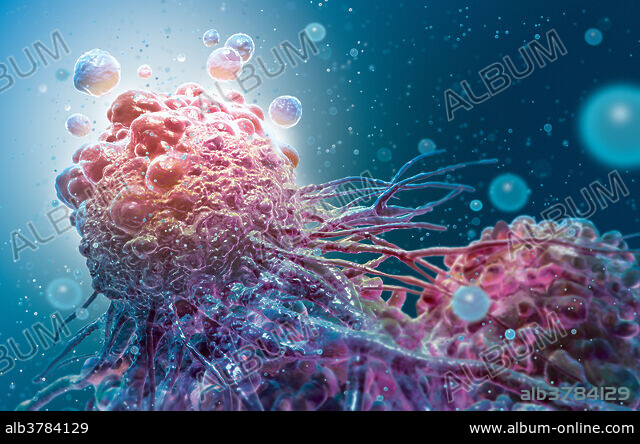The image depicts a possibly computer-generated, undersea creature prominently situated in the top left corner of a dark blue, bubble-filled background. The creature, resembling a jellyfish, is a large, spherical, rough-textured organism with a dark pink to light pink gradient. Multiple tentacle-like or branch-like structures extend from its underside, adding to its dynamic appearance. Surrounding this primary creature are numerous bubbles of different sizes, some translucent and others in shades of pink, white, and blue, contributing to an underwater atmosphere. The image features a watermark of the word "ALBUM" stamped repeatedly across it. At the bottom of the image, there's a black band with the text "ALB3784129" on the left side and "www.albumonline.com" on the right.